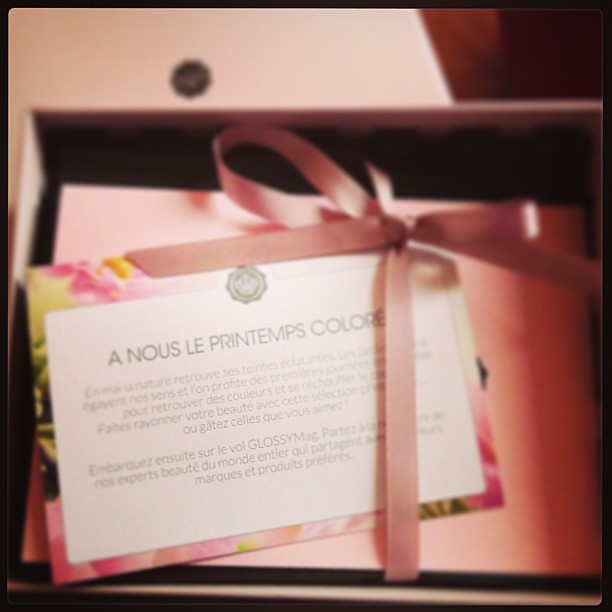The image features a detailed view of a gift box. The primary object is a pink box adorned with a neatly tied pink ribbon and an elegant bow. This pink box, laying flat and centrally positioned, is nestled inside a larger open box. Accompanying the pink box is a floral card with pink, green, and yellow trim against a white background. The card contains text written in a foreign language, possibly French, with phrases like "Anus Lee Printemps," though the exact meaning isn't entirely clear. The open larger box, which appears pink or white, has its lid placed underneath it, revealing the gift inside. While the exact setting of the image is ambiguous, it seems to be taken indoors, possibly in a gift shop or as a snapshot of a recently received gift. The scene is bright, suggesting it might be daytime.